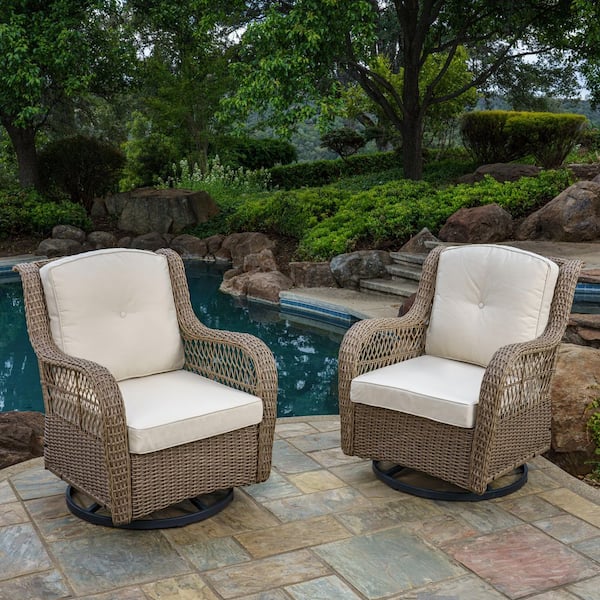The image captures a serene backyard oasis featuring a naturalistic in-ground pool flanked by intricate rock formations and lush greenery. Verdant foliage, trees, and rolling green hills form a picturesque backdrop, making the scene feel intimately connected with nature. In the foreground, there is a stone patio with two identical, wicker swivel lounge chairs. These chairs, adorned with cream-colored cushions, are positioned at a slight angle to each other, overlooking the tranquil pool. Steps lead from the patio down into the pool, and reflections of the surrounding trees dance on the water's surface. The stone patio itself features a blend of colors including blue, pink, white, and beige, adding to the aesthetic charm. The absence of any people or lettering and the presence of flowers scattered throughout the background contribute to the peaceful and luxurious ambiance, making it an inviting space for relaxation and contemplation.